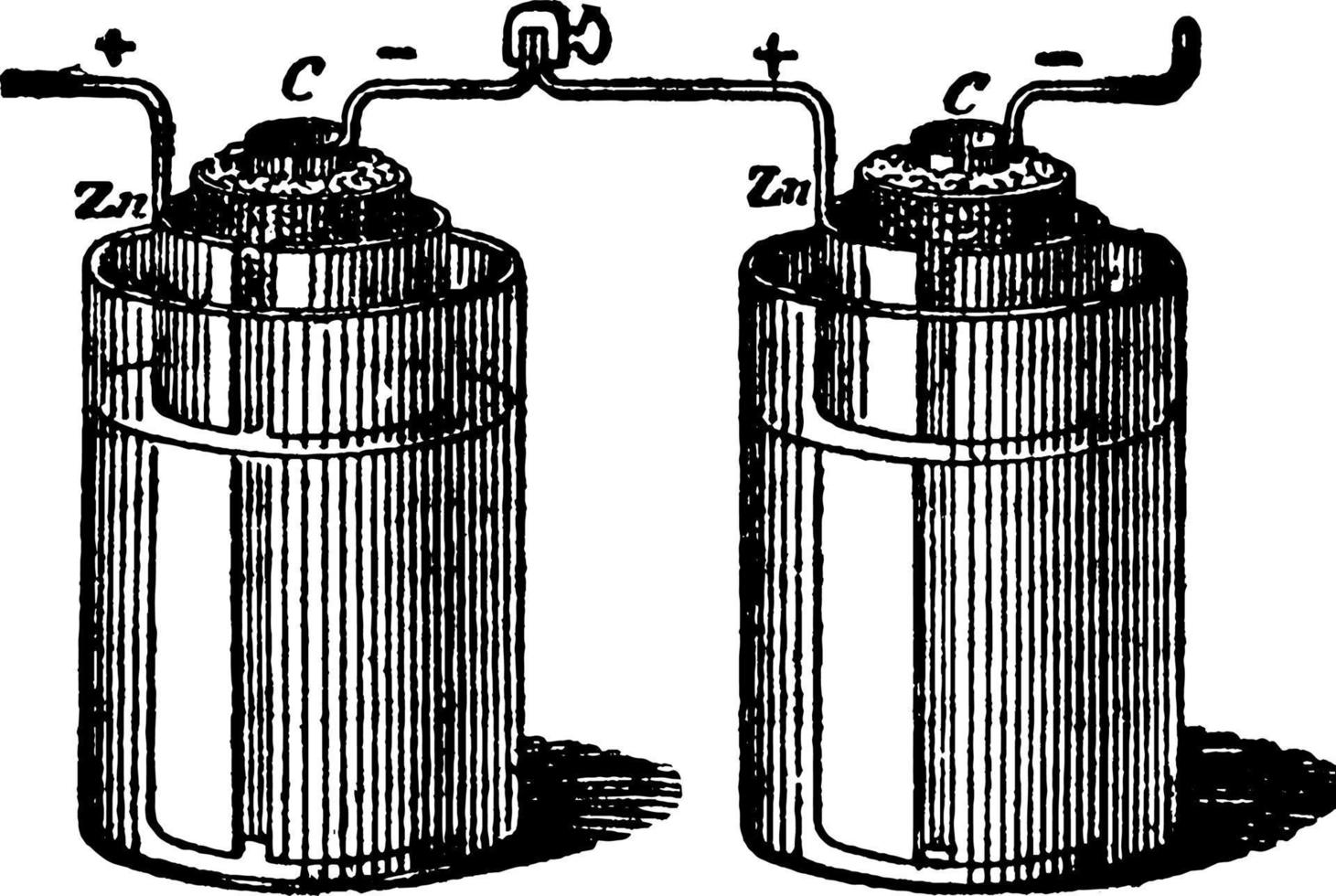The image depicts a detailed black-and-white computer-drawn illustration of two cylindrical batteries connected by a metallic wire. The batteries are labeled with various symbols and letters. Around the rim of one battery, there is a marking "Z" with a plus sign located just above a small wire extending from it. To the right of this, the other battery features markings "C" and a minus sign. The two batteries are interconnected by a twisty valve mechanism, and there are additional wires coming out of both batteries. Underneath the wiring, there are inscriptions "Z+" and "C-". A semicircular shadow from the batteries is visible on the ground, adding a realistic touch to the illustration.